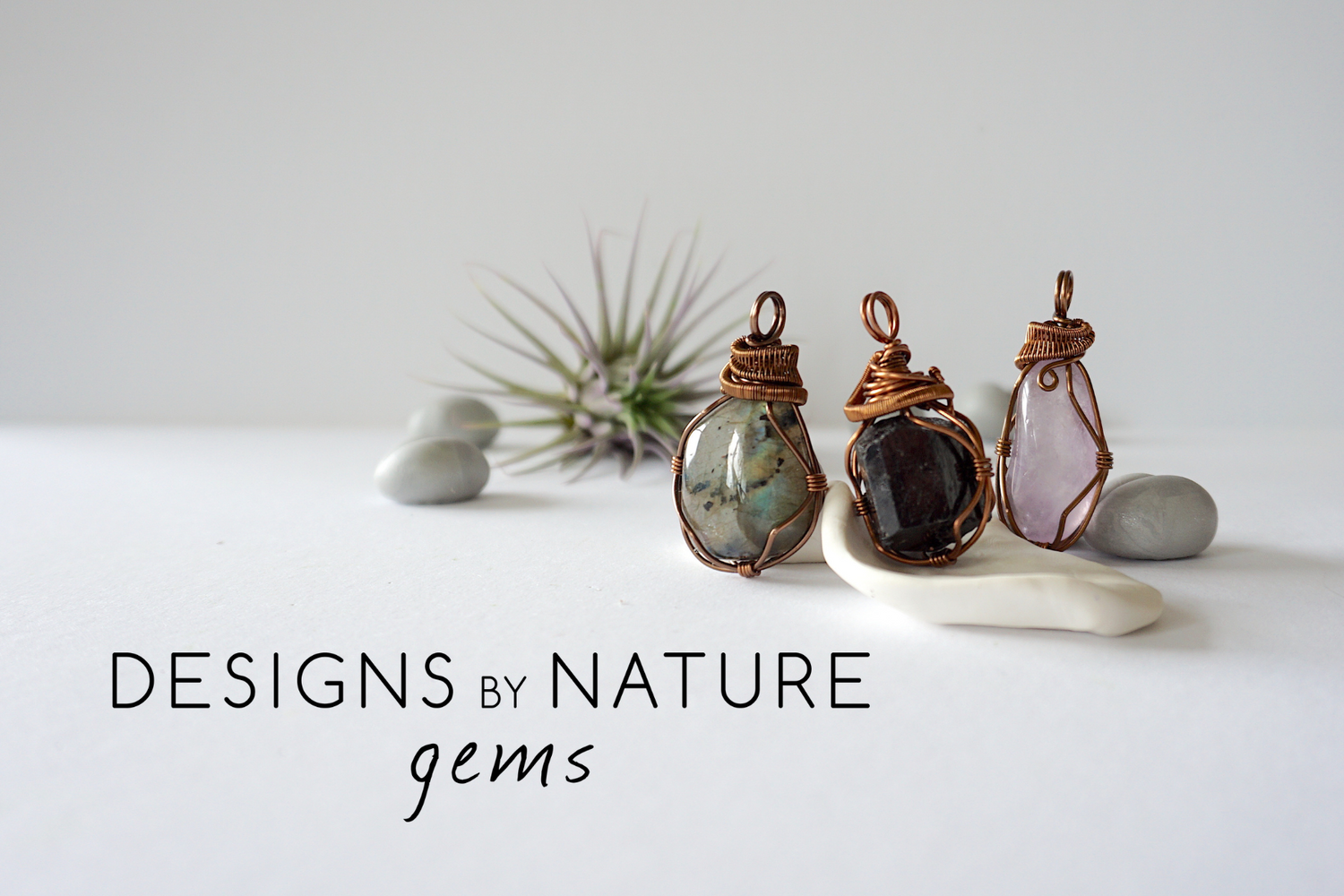This horizontal rectangular photograph, which appears to be an advertisement, prominently features three naturally shaped crystal pendants in a clean and light setting. The caption at the bottom left reads "DESIGNS BY NATURE" in thin black capital letters, and underneath it, "gems" in lowercase script. The three pendants, each meticulously wrapped in copper wire, stand upright with loops at the top to attach to a necklace or bracelet. The first pendant is an irregularly shaped green stone, the second is a polished black stone placed atop a white seashell, and the third is a soft pink or light purple gem. The scene is set against a white surface and background, complemented by a spiny plant and several small white and olive green pebbles, adding to the naturalistic theme of the design.